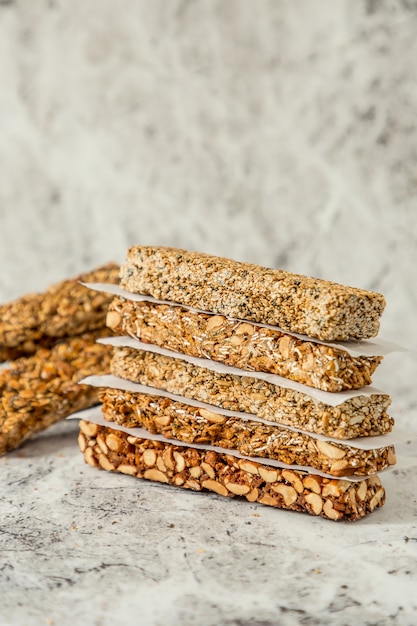The image showcases a close-up of handmade granola bars, arranged meticulously on a marbled gray and black countertop that blends seamlessly with the similarly styled backsplash in the background. The food items are cut into rectangular bars, distinctly separated by thin pieces of white wax paper. There are five granola bars stacked vertically in the center of the image, with two additional bars lying side by side on the countertop behind the stack. These bars feature a varied texture and coloration, displaying different shades of brown, and are embedded with flat, light-to-dark-colored nuts and grains. The overall presentation implies a promotional or recipe shot, highlighting the handcrafted nature of the granola bars.